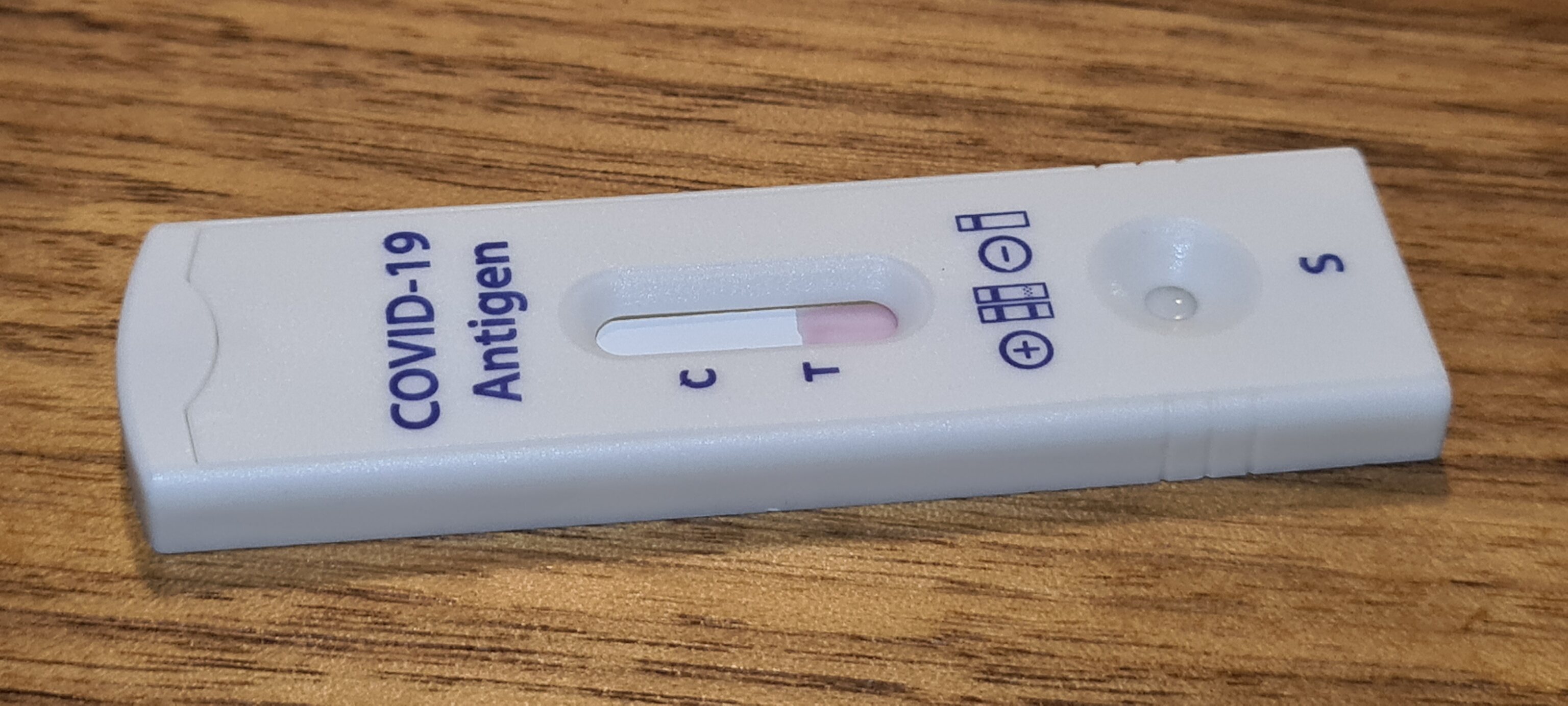The image depicts a single COVID-19 antigen test placed in the center of a wooden table. The test, characterized by its white body and blue lettering, prominently displays the text "COVID-19 antigen." There is a "CT" marking on the test, along with various symbols and an "S" indicator. The presence of a faint pink line suggests a possible positive result, although the absence of a second line makes it difficult to confirm. The overall design of the test includes small wedges. The background showcases the textured pattern of the wooden table, which may be faux wood.